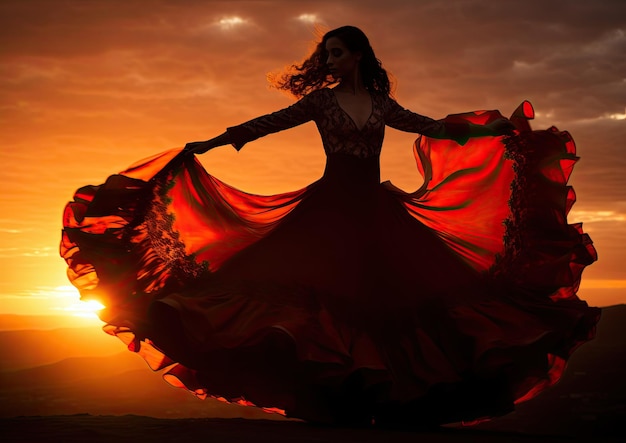In this captivating outdoor photo, a woman is captured mid-spin in a striking red flamenco-style dress at sunset. The dress features elaborate, frilly edges that she holds outstretched, creating a dramatic, wing-like effect as it flares around her. Her long hair, slightly twirling from her movement, hints at her turning position. The red dress, low-cut across her chest, is illuminated from behind by the golden rays of the setting sun, casting her into a shadowy silhouette. The sky, filled with orange and golden clouds, contrasts beautifully with the dark mountains visible in the background, adding depth to the scene. The sun, nestled near the horizon, bathes the entire image in a fiery gold light, enhancing the ethereal quality of the photograph.